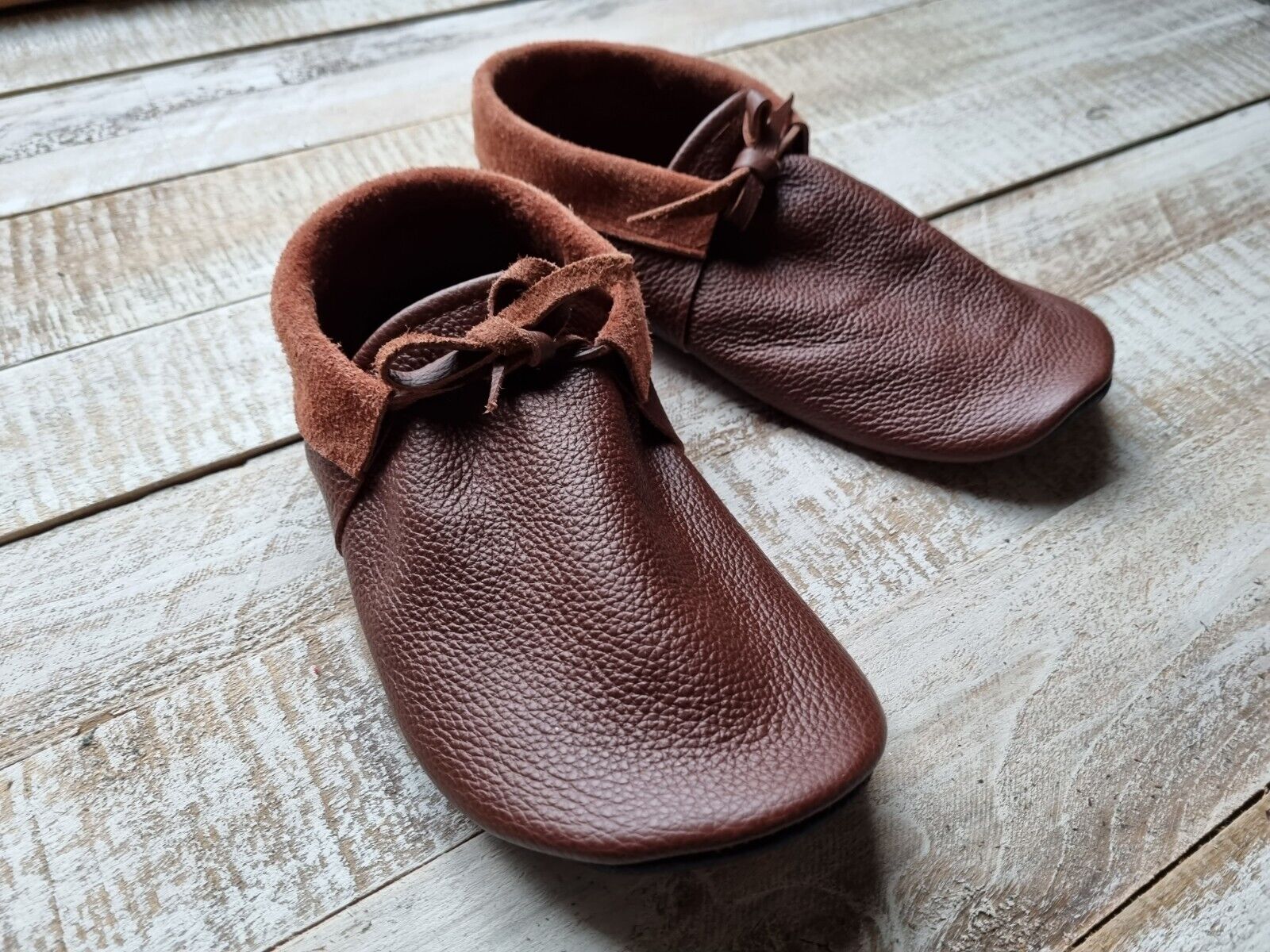This photograph showcases a pair of handmade baby moccasins made of genuine brown leather, prominently placed on an unpolished, grayish wooden floor. The moccasins exude a minimalist design, featuring a soft suede lining inside and around the top that folds down to ensure comfort for a baby's ankles. The leather ties, seamlessly integrated from the same material as the shoes, secure the moccasins, which lack a typical tongue and sole, giving them a seamless and adaptable form. The lighting in the image is soft and even, accentuating the natural textures and imperfections of both the shoes and the wooden planks beneath them. The floor, with its uneven patterns and natural color, complements the rustic, handcrafted feel of the moccasins, creating a professional yet intimate product photo.